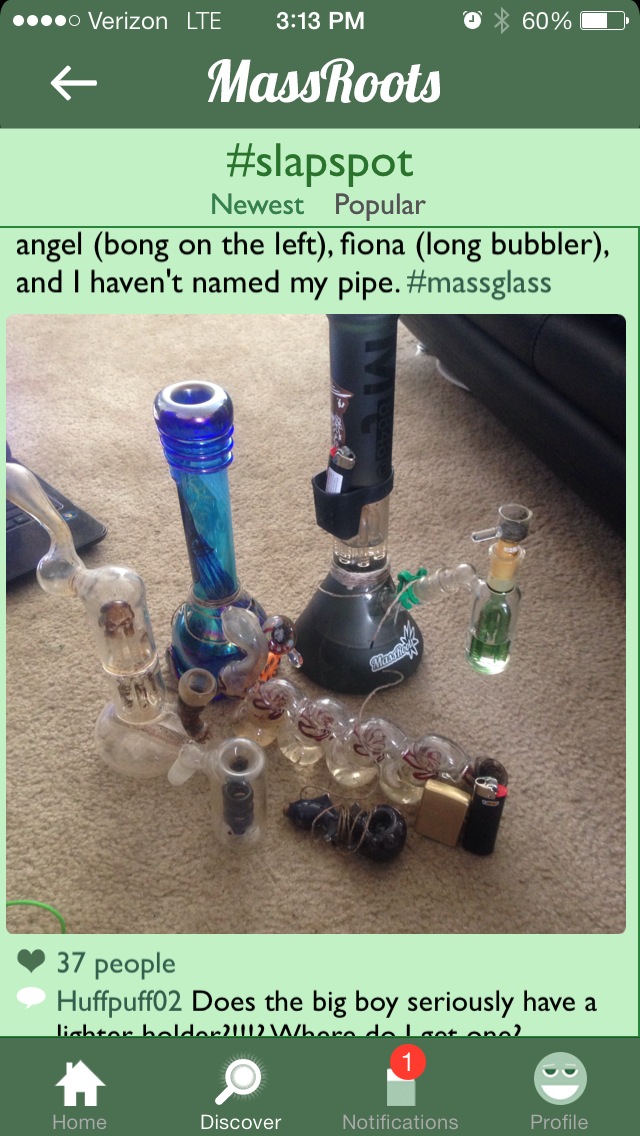This is a colour photograph of a smartphone screenshot, showcasing a web page optimized for mobile viewing. At the top, the phone's user interface displays a green border labeled Verizon LTE, the time (3:13 PM), and a battery icon showing 60% remaining. Below this, there's a left arrow beside the text "Mass Roots." Further down, there's another green section with the header "#SlapSpot, newest popular." The description reads, "Angel Bong on the left, Fiona Long Bubbler, and I haven't named my pipe. #MassGlass." 

The main part of the image exhibits various glass smoking paraphernalia on a beige carpet—one blue bong with a round bottom and long stem, and a black bong in the center. To the left, there appears to be a clear pipe among other glass objects likely part of the collection. At the bottom left-hand corner, you see the text "37 people like that," along with a comment from user HumpPuff02 reading, "Does the big boy seriously have..." (the rest of the message is cut off). The bottom green area features mobile controls: icons for home, discover, notifications (with a red circle and the number one), and a profile symbol.